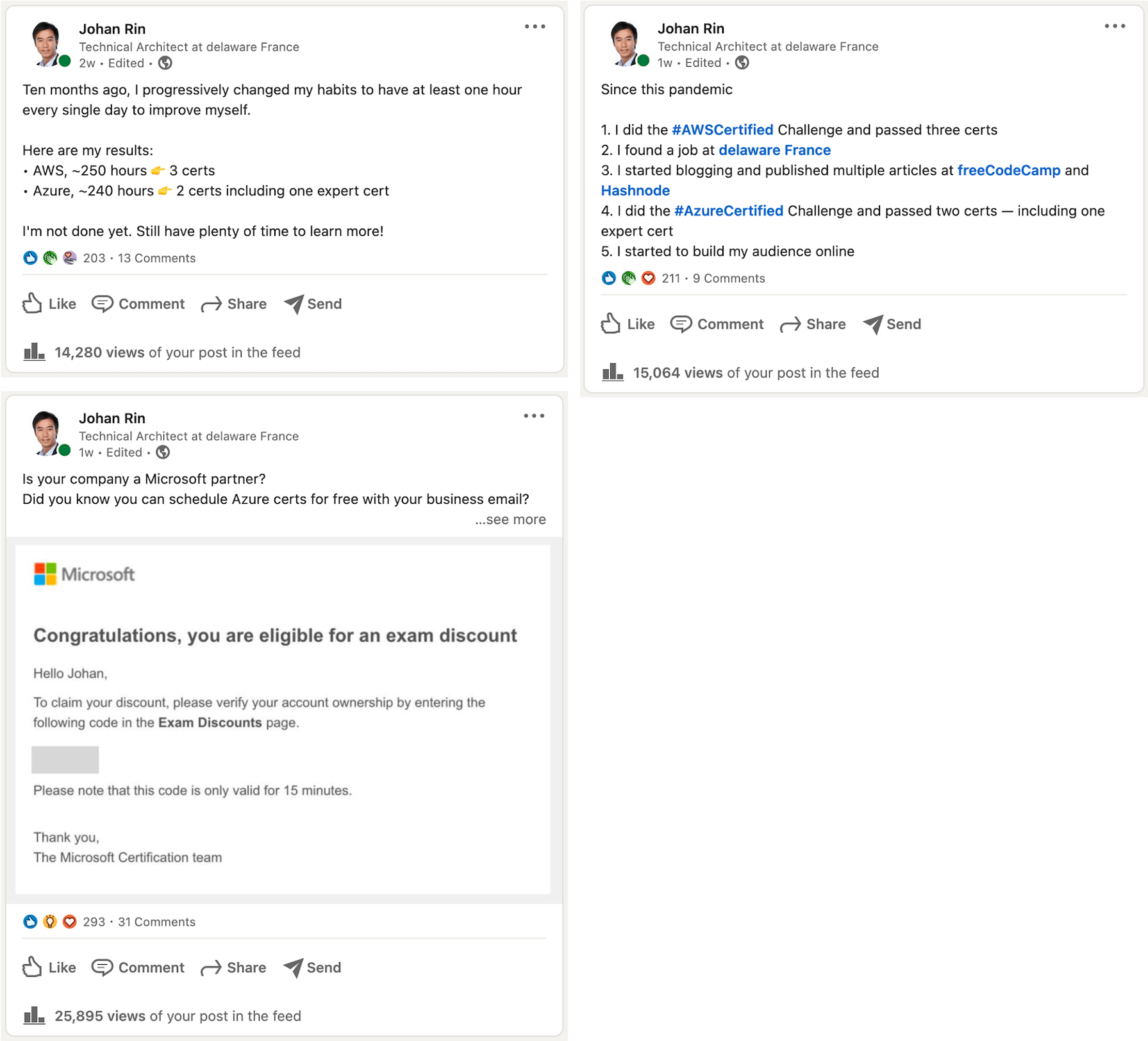Three detailed screenshots prominently feature John Johan Wren, who displays a profile picture of a man in a suit with a green status dot. Each screenshot reflects various stages of his updates over time. 

In the first screenshot, titled "2W edited," John shares a reflective post detailing his journey over the last 10 months. He explains how he has progressively changed his habits to dedicate at least one hour daily to self-improvement and celebrates his ongoing progress. The post ends on an optimistic note, emphasizing that he still has plenty of time to learn more. The image includes social media interaction icons: like, comment, share, and send.

The second screenshot, labeled "1W edited," features John's professional accomplishments. In this update, he inquires, "Is your company a Microsoft partner?" The post includes a "See more" section that reveals that John has recently received congratulations for being eligible for an exam discount, signed off by the Microsoft Certification Team.

The third screenshot, also "1W edited," addresses how John has adapted during the pandemic. This post includes numbered bullet points from one to five, elaborating on various pieces of information related to his experiences and actions taken during this time.

Each screenshot features consistent graphical elements: a globe image and three horizontal dots aligned to the far right, providing more options or additional information when clicked.